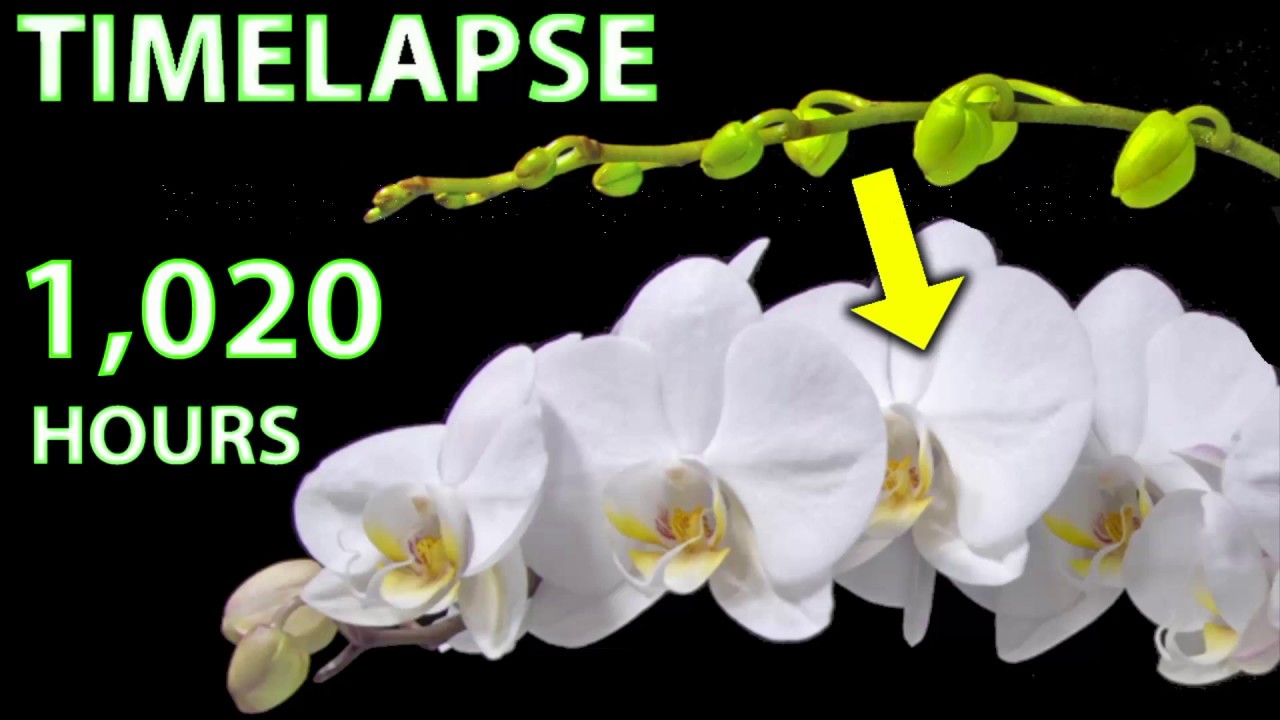This image, likely a frame from the beginning of a YouTube time-lapse video, showcases a stunning transformation of flowers from seeds. Against a black background, the upper left corner of the image features the word "Time-lapse" in green neon letters, accompanied by "1020 hours" directly below. The visual centerpiece is a branch of approximately six white orchids with intricate yellow centers, some showing subtle hints of pink or purple. The branch begins in the lower right corner, extending out towards the lower left, where a few buds remain unopened. Above this flowering branch, a separate green stem holds small green buds that have yet to bloom. This stem, originally green, has turned brown over time, illustrating the progression captured by the time-lapse. An illustrative yellow arrow points from the green buds, now transformed, highlighting the transition into the beautiful white flowers with vivid centers.